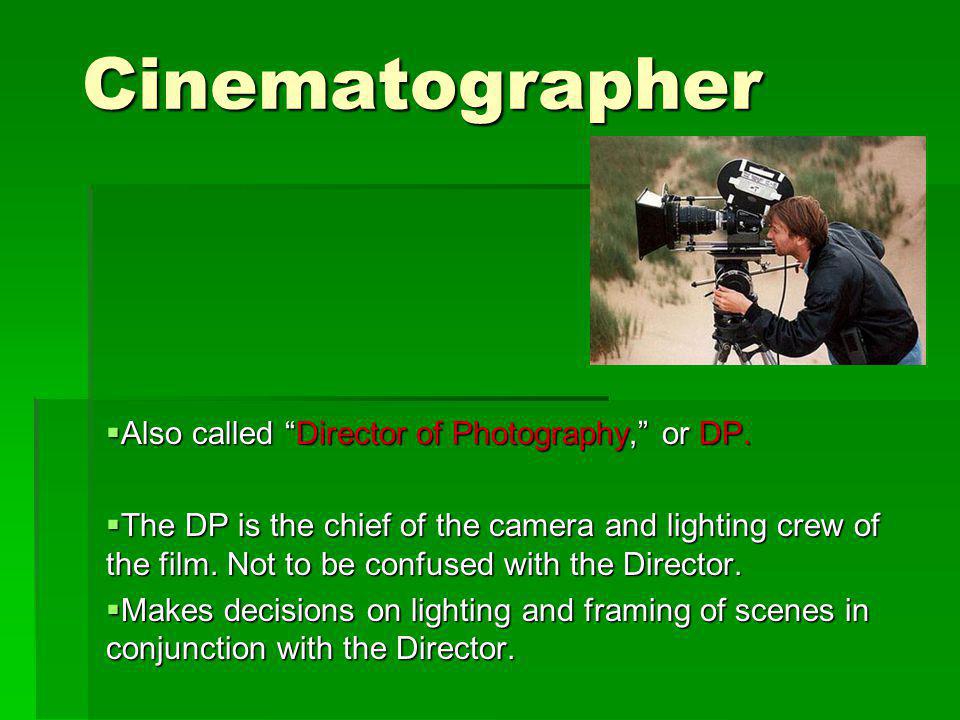The image is an informational slide, likely from a PowerPoint presentation, featuring a lime green background with a title, a photo, and explanatory text. At the top, "Cinematographer" is clearly displayed in yellowish-white text. Below it, a small photo justified to the right depicts an adult white male with mid-length brown hair, wearing a black jacket and jeans, operating a large, seemingly outdated camera with black parts and a black lens. The background of the photo suggests a dry area with sand and trees. Beneath the photo, white text in a bordered section reads: “Also called ‘Director of Photography’ or ‘DP’” with "Director of Photography" and "DP" highlighted in red. Further down, it explains that the DP is the chief of the camera and lighting crew on a film, a role not to be confused with the director, and elaborates that the DP makes decisions on the lighting and framing of scenes in collaboration with the director.